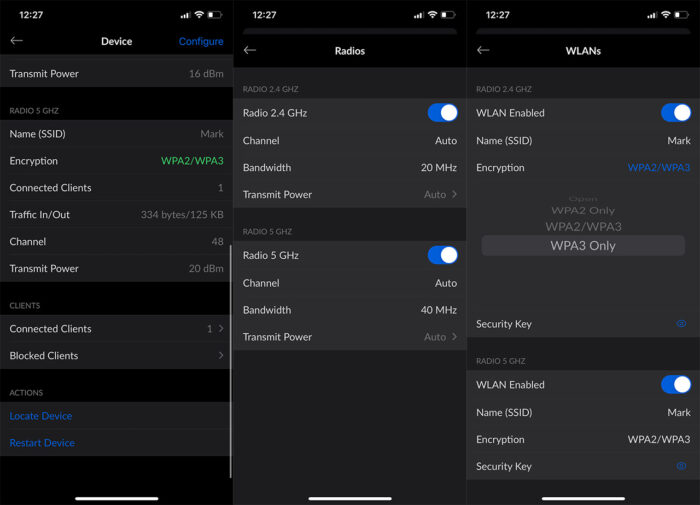### Descriptive Image Caption:

This image is a composite of three phone screenshots, each representing a different page of a device management interface. The screenshots are organized into three distinct columns with a timestamp of 12:27.

**First Column: Device Page**
- **Heading: Transmit Power**
- **Subheading: Radio 5GHz**
  - **SSID (Name of WLAN)**
  - **Encryption Methods**
  - **Connected Clients**
  - **Traffic In and Out**
  - **Channel Info**
  - **Transmit Power Levels**
- **Heading: Clients**
  - **Connected Clients**
  - **Blocked Clients**
- **Heading: Actions**
  - **Locate Device**
  - **Restart Device**

**Second Column: Radio Screen Page**
- **Heading: Radio 2.4 GHz**
  - **Radio is turned ON**
  - **Channel: Auto**
  - **Bandwidth: 20 MHz**
  - **Transmit Power: Auto**
- **Heading: Radio 5 GHz**
  - **Radio is turned ON**
  - **Channel: Auto**
  - **Bandwidth: 40 MHz**
  - **Transmit Power: Auto**

**Third Column: WLANS Page**
- **Section: Radio 2.4 GHz**
  - **WLAN: Enabled and turned ON**
  - **SSID (Name): Mark**
  - **Encryption: WPA2 / WPA3**
  - **Security Key: Present**

- **Section: Radio 5 GHz**
  - **WLAN: Enabled and turned ON**
  - **SSID (Name): Mark**
  - **Encryption: WPA2 / WPA3**
  - **Security Key: Present**

This detailed breakdown highlights the key settings and status information related to the wireless radios and network security configurations for both the 2.4 GHz and 5 GHz bands.